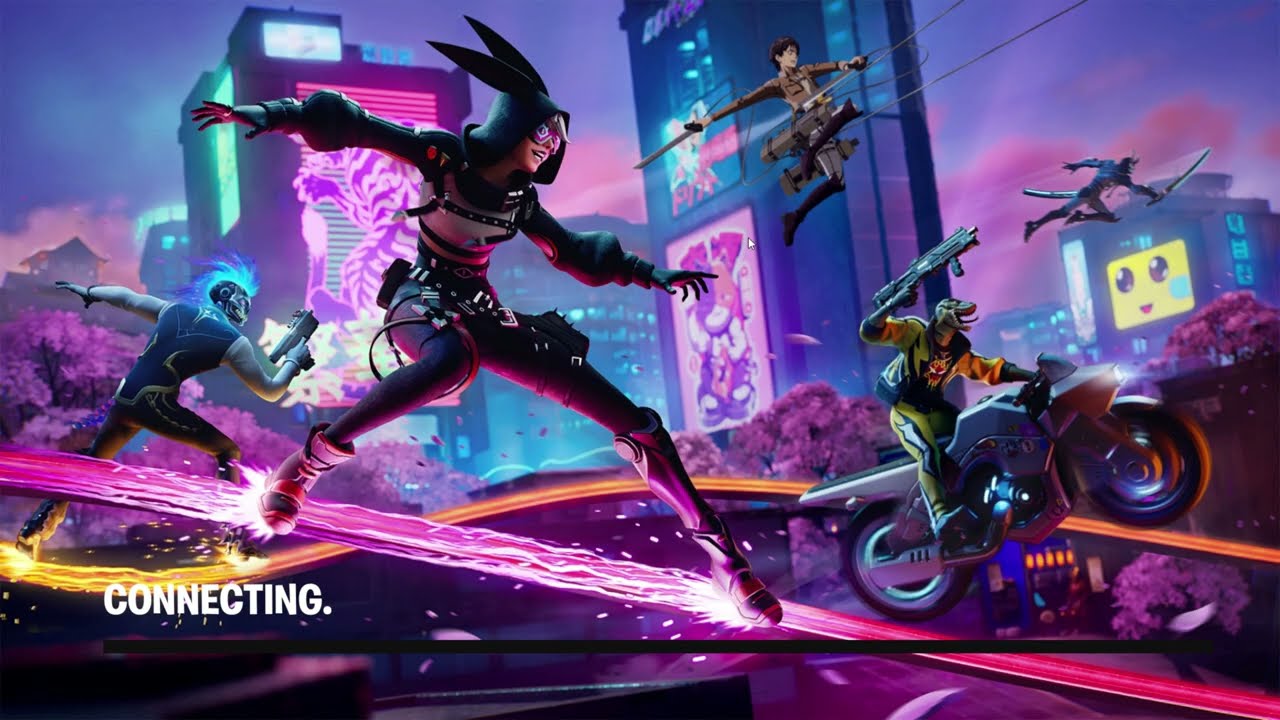The image appears to be the futuristic loading screen of a video game, possibly Fortnite, characterized by its vivid neon and cyberpunk aesthetics reminiscent of a Tokyo cityscape. The lower left corner features the word "CONNECTING." in all uppercase white letters. The scene is set against a backdrop of skyscrapers adorned with neon signage, including a notable smiley face on one of the buildings. The environment is primarily hued in shades of purple, blue, lavender, and pink. 

In the foreground, a prominent character wearing a suit of armor with a two-eared black helmet surfs on a pink stream of electricity, adorned with wires and attachments on their legs. Right behind, a blue-mohawked character handles a weapon as they navigate a yellow electric bolt. Further along, a lizard-faced figure brandishes a machine gun while riding a motorcycle in mid-air. High above, a small figure with a sword flies through the sky, seemingly suspended without support. Another character, resembling a dog, rides a light energy vehicle, though they carry no visible weaponry. Lastly, a human figure with a harness and a sword is seen soaring through the air, tethered by strings extending off-screen. Each character is rendered with unique skins suggestive of the game's customizable features, adding to the intricate art style of this dynamic, electricity-filled tableau.